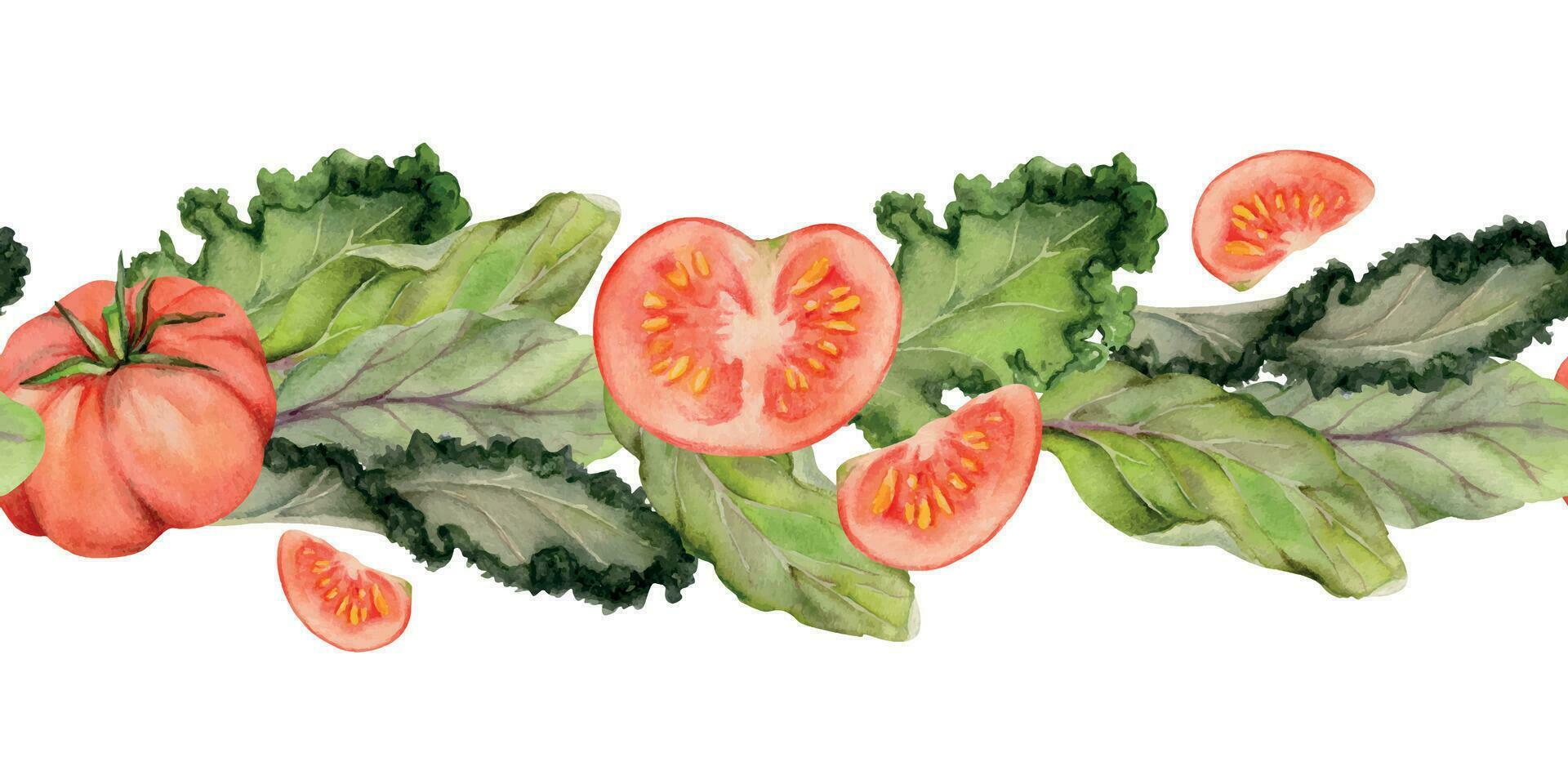This image is a detailed painting of fresh lettuce leaves and tomatoes, set against a stark white background. In the composition, a fully formed tomato with its green stem prominently protrudes on the far left. This tomato is depicted in a reddish-pink hue and lies atop a bed of lush green lettuce. Just to the right of the whole tomato is a quarter slice of tomato, displaying its yellow seeds. Centrally positioned in the picture, a halved tomato reveals its internal structure and seeds. Scattered around this central element are three additional tomato quarters, with one located to the bottom right, showing off its seeds as well, and another upside-down piece floating near the right edge above the cabbage. The lettuce, characterized by its vibrant shades of dark and light green, extends across the entire painting, contributing a fresh and appetizing appearance to the scene. The harmonious blend of green, red, and yellow tones against the white background emphasizes the rich colors and textures of the vegetables. The artwork appears to be rendered using either colored pencils or watercolors, giving it a realistic yet delicate feel.